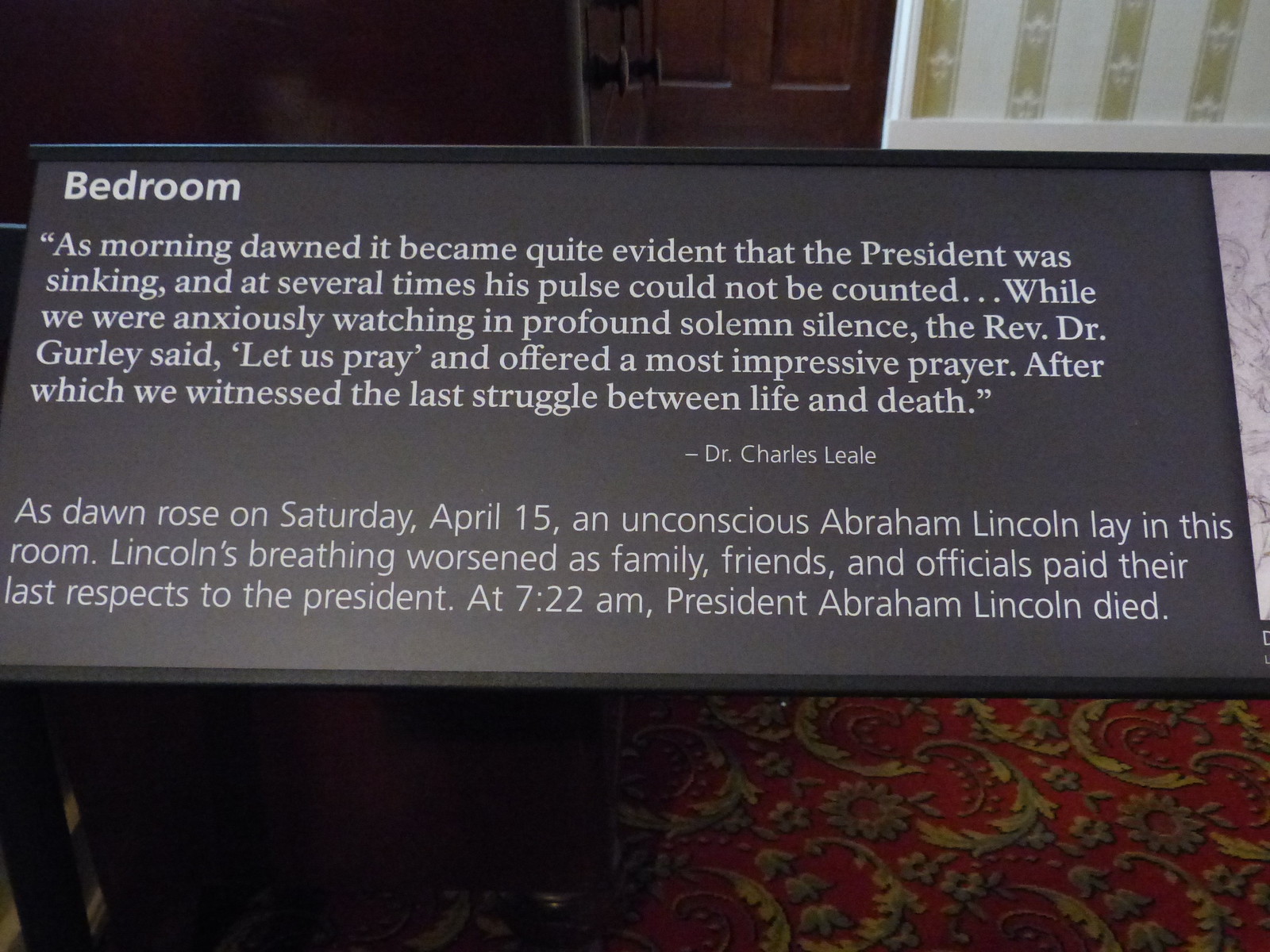This photograph captures a museum exhibit placard with a gray background and white text, prominently displaying the word "Bedroom." The placard features a quote by Dr. Charles Leale, describing the final moments of President Abraham Lincoln's life: "As morning dawned it became quite evident that the president was sinking and at several times his pulse could not be counted. While we were anxiously watching in profound solemn silence the Reverend Dr. Gurley said, 'Let us pray,' and offered a most impressive prayer, after which we witnessed the last struggle between life and death." Below the quote, the placard explains that on the morning of April 15th, an unconscious Abraham Lincoln lay in this room, his breathing worsening as family, friends, and officials paid their last respects. At 7:22 a.m., President Abraham Lincoln passed away.

The gray placard is set against a backdrop that includes a red and green carpet in the bottom right corner, suggesting the historical setting of the exhibit. The surrounding cabinetry hints at an indoor museum environment, with the placard being the focal point of the image.